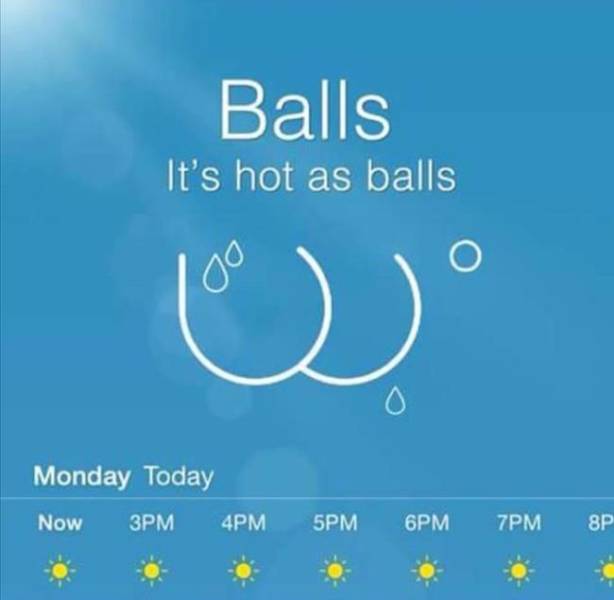The image depicts a weather forecast with a solid blue background reminiscent of the sky. Centered at the top is the bold word "BALLS" followed by the phrase "it's hot as balls" in smaller text directly below. Beneath this, two semicircles outlined in white form partial shapes resembling balls. The left semicircle contains two raindrops, while the right semicircle features a circle at its upper right and another raindrop just below it.

At the bottom of the image, the text "Monday today" appears on the left side. Below, a timeline runs across the image, starting with "NOW" followed by hourly markers from "3PM" to "8PM," though the last "PM" is partially cut off. Directly under each time marker, a yellow sun icon with radiating lines indicates sunny weather throughout the day. The overall color scheme consists of white, blue, and yellow elements, enhancing the visual representation of a sunny, hot day.